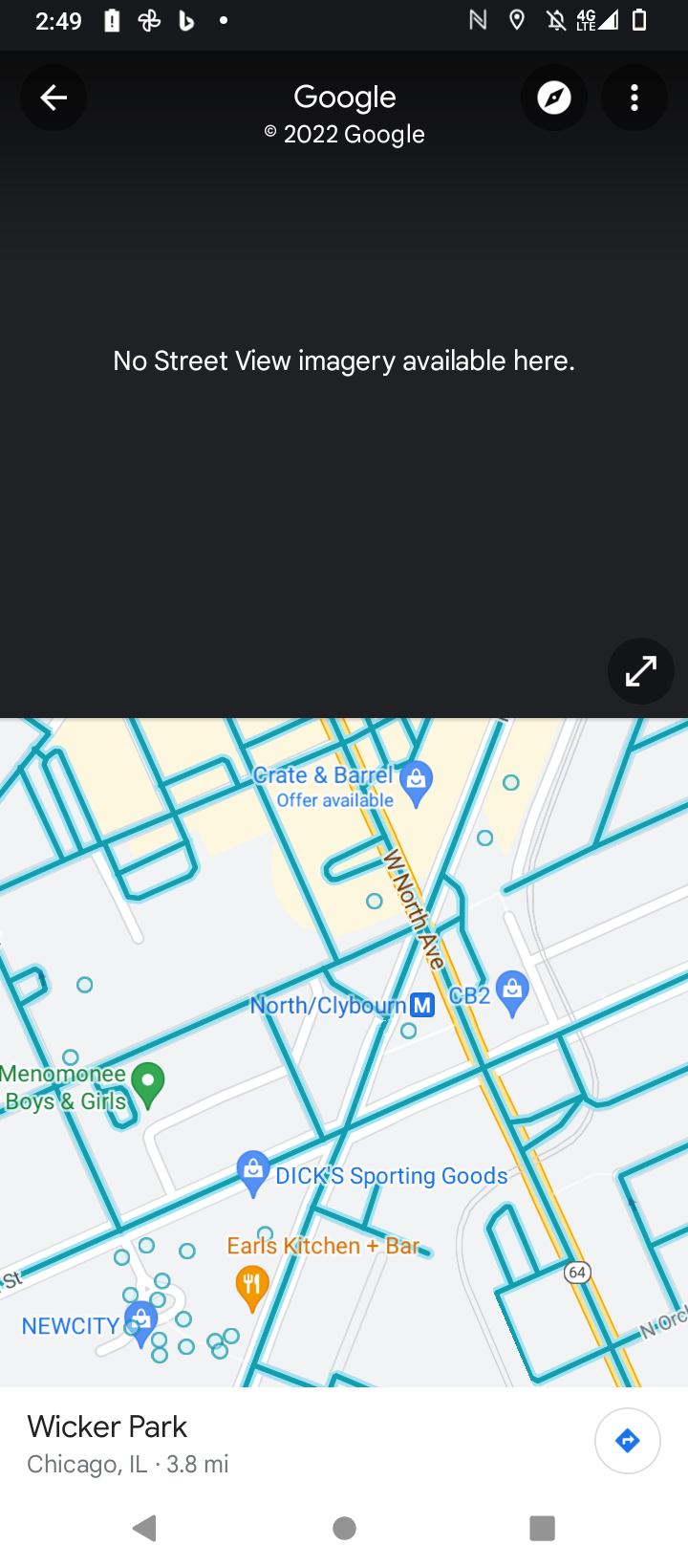This is a detailed Google Maps snapshot of Wicker Park in Chicago, Illinois, captured in 2022. The image reveals that no Street View imagery is available for this specific area. The map is a bird's eye view showing the streets and their names rather than a satellite view. 

The map highlights various stores and landmarks around Wicker Park:

- At the top, it indicates a promotional offer for Crate & Barrel in blue text.
- North Clybourn, a transportation stop, intersects with West North Avenue (Route 64).
- CB2, another popular shopping location, is marked nearby.
- Dick's Sporting Goods is also featured, although its exact street is not listed.
- East of the area, there is 'Earl's Kitchen + Bar' and a region referred to as 'New City'.
- Additional locations marked include 'Bowls and Memoir', and 'Me, Me, Boys and Girls'.

The map effectively shows a dense concentration of commercial activity in Wicker Park, providing a snapshot of the area's bustling retail scene.